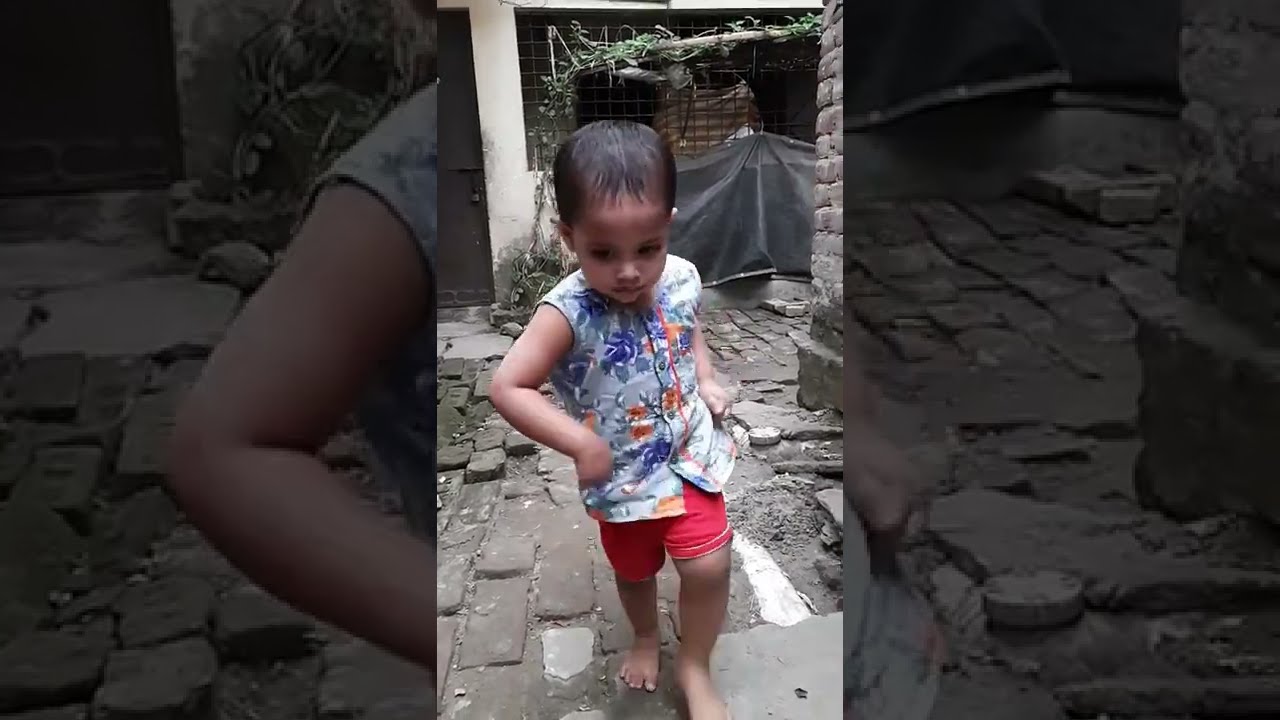This vertical color photograph captures a young toddler with black hair, wearing a sleeveless, multicolored floral shirt, and red shorts. The child, who is barefoot, is walking towards the camera on gray stone paving, with the right arm extended forward and the left arm backwards. The setting appears to be an alley or patio, with a stone wall on the right and a trellis with green plants or vines. The background features a white wall and a black door, with natural light illuminating the scene, emphasizing the contrast between the vibrant colors of the child’s clothing and the muted tones of the surrounding environment.